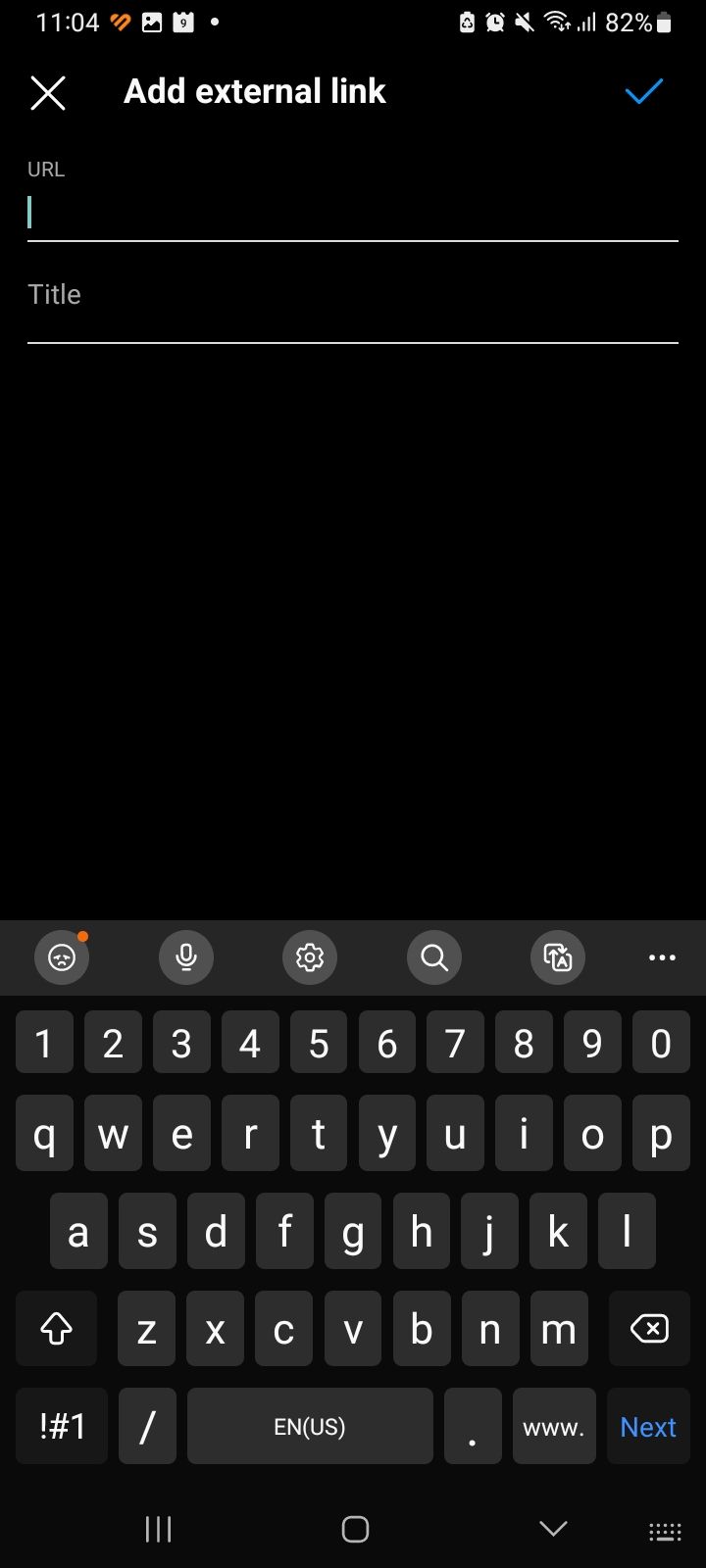This screenshot, taken from an Android device in dark mode, captures an interface element for adding an external link. The screen displays a "Add External Link" header, with a white "X" for closing the dialog on the upper left and a blue checkmark on the upper right for confirming the action. Below this header, there are two clear entry fields labeled "URL" and "Title," both awaiting input. The layout features a substantial blank space, approximately the size of the keyboard shown at the bottom of the screen.

The virtual keyboard covers nearly half of the lower portion of the display. It includes buttons for emojis, a microphone, settings (gear icon), and search functionality. Above the primary QWERTY keyboard, there is a horizontal line of numbers ranging from 1 to 9, followed by 0. The keyboard keys are displayed in white text against a dark gray background, contributing to the overall dark theme of the interface.